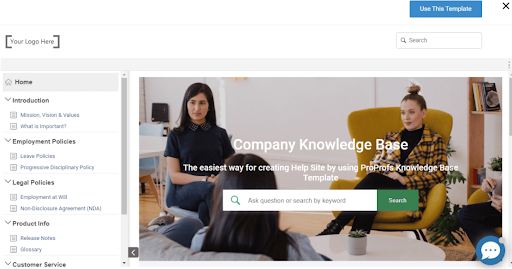This advertisement is designed to attract individuals interested in creating their own website. In the top left corner, a placeholder text "Your Logo Here" suggests easy customization options for branding. The top right corner features a call-to-action button labeled "Use This Template," inviting users to get started quickly.

On the left side of the webpage template, there is a navigation pane with drop-down options including Introduction, Employment Policies, Legal Policies, Product Info, and Customer Service, providing a comprehensive structure for any professional website.

The centerpiece of the advertisement showcases an image of two women seated and facing an audience or other women, under the header "Company Knowledge Base." The headline states, "The easiest way for creating a help site by using ProProf's Knowledge Base template," emphasizing the user-friendly nature of the product.

Directly below the image, a search bar prompts with "Ask Question or Search by Keyword," accompanied by a green magnifying glass and a green search button, enhancing the intuitive search functionality.

In the bottom left corner, a speech bubble icon with three dots suggests the availability of live chat support to assist users in navigating the website. The entire layout is devoid of any animal imagery and maintains a professional aesthetic, clearly targeted towards business users.